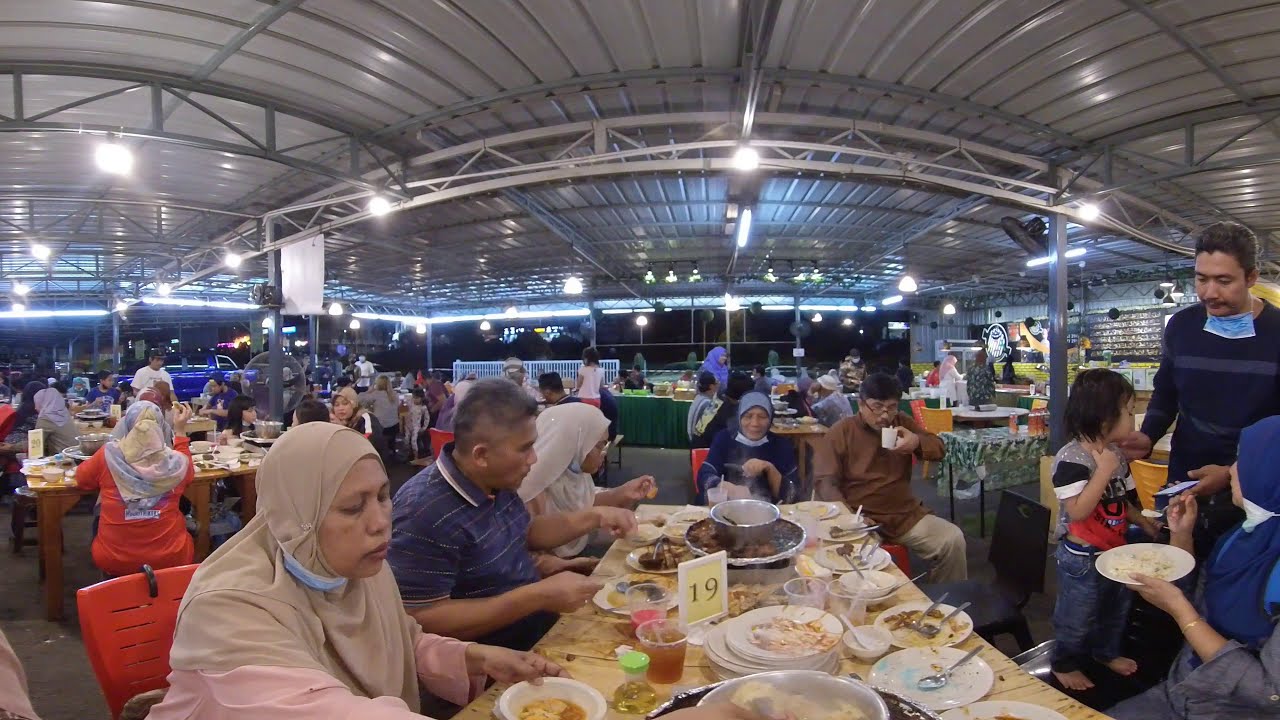The image depicts a bustling, open-air restaurant with a large, horizontal, and rectangular layout. The scene is lively, with numerous people sitting at tables, enjoying their meals together. The restaurant's ceiling is made of gray-silver corrugated metal, with steel girders running across it and white lights attached. 

In the center, a large, unfinished wooden table stands out, marked with a plaque card indicating the number "19." Surrounding this table is a family of about eight to nine people, with at least four women wearing hijabs, reflecting the cultural diversity of the patrons. The diners appear to be of Middle Eastern or South Asian descent, with a mix of men and women, all engaged in communal dining. 

At the far end of the restaurant, there's an ordering area with a menu displayed on a black wall. A buffet table draped with a green curtain is also visible. The fisheye lens effect creates an extreme curvature in the image, adding a unique visual distortion. The night setting is evidenced by the lights on the buildings seen through the open-air sides of the restaurant. Overall, the scene captures a warm, communal dining experience in a culturally rich and diverse setting.